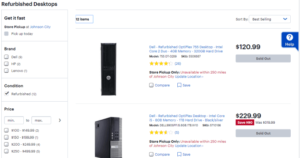This image showcases a webpage featuring two desktop towers from a well-known manufacturer of laptops and desktops. The image is small and not zoomed in, making details challenging to discern. 

The first desktop tower is positioned front-facing, has a sleek black design, and boasts a rating of approximately 4.2 to 4.5 stars based on a few hundred reviews. It is priced at $120.99 USD. 

The second desktop tower is displayed side-facing and is lighter in appearance compared to the first. It has garnered around a 4-star rating with only double-digit reviews and is priced at $229.99 USD. 

Beneath each price, there appears to be a deal highlighted within a red box, although the specific text is not visible. Adjacent to this highlighted box, there's some grey-colored text likely indicating the original prices before the discount, though the exact figures are indistinguishable. Both desktop options include an "Add to Cart" button beneath their respective prices. 

In the top right corner of the page, there is a blue "Help" button for customer assistance. On the left-hand side, a variety of filters are available to help users refine their search.